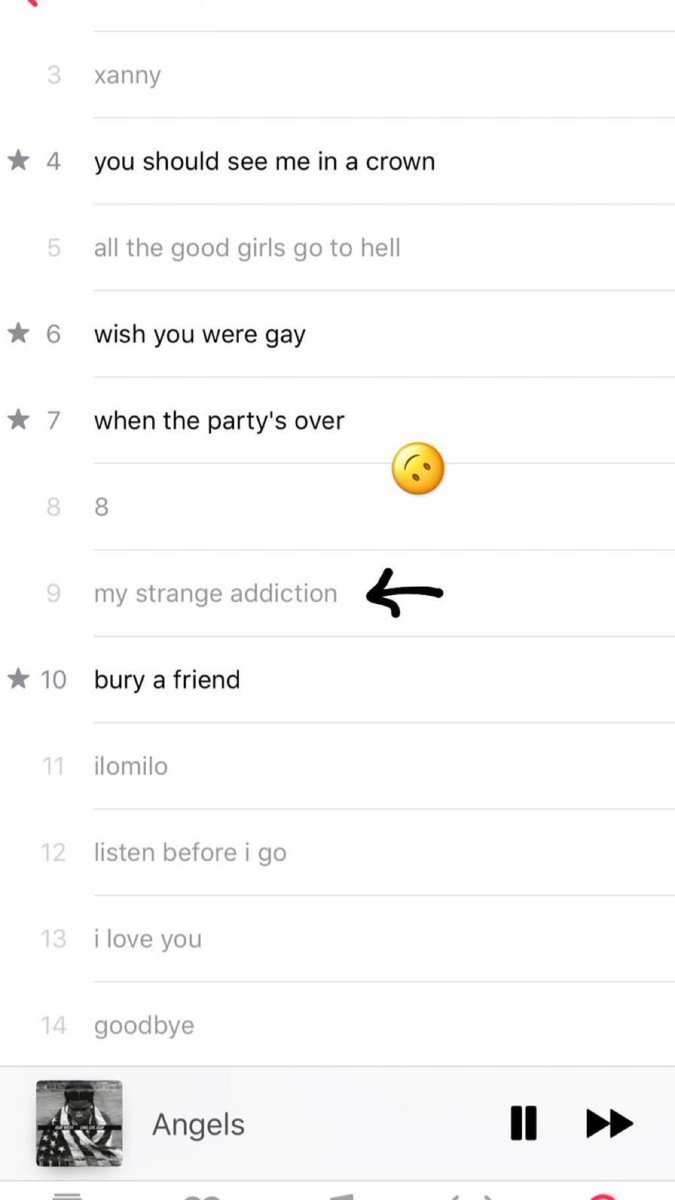A screenshot of a Spotify playlist is displayed on a clean white background, with song titles separated by thin gray lines. In the top-left corner, a small red marking is visible. Just below this marking, the playlist begins: 

1. "Xanny" 
2. "you should see me in a crown" (indicated with a star to the left)
3. "all the good girls go to hell"
4. "wish you were gay" (also marked with a star)
5. "when the party's over" (marked with a star)
6. "8"
7. "my strange addiction" (highlighted by a black arrow pointed towards it)
8. "bury a friend" (starred)
9. "ilomilo"
10. "listen before I go"
11. "I love you"
12. "goodbye"

Located beneath these titles, the term "angels" is mentioned, accompanied by an album cover image to the left, depicting a Black girl draped in a flag. To the right of this image are the playback controls: a pause button and a fast forward button.

Additionally, between the seventh and eighth tracks on the list, a yellow smiley face emoticon is positioned, tilting slightly at an 80-degree angle.